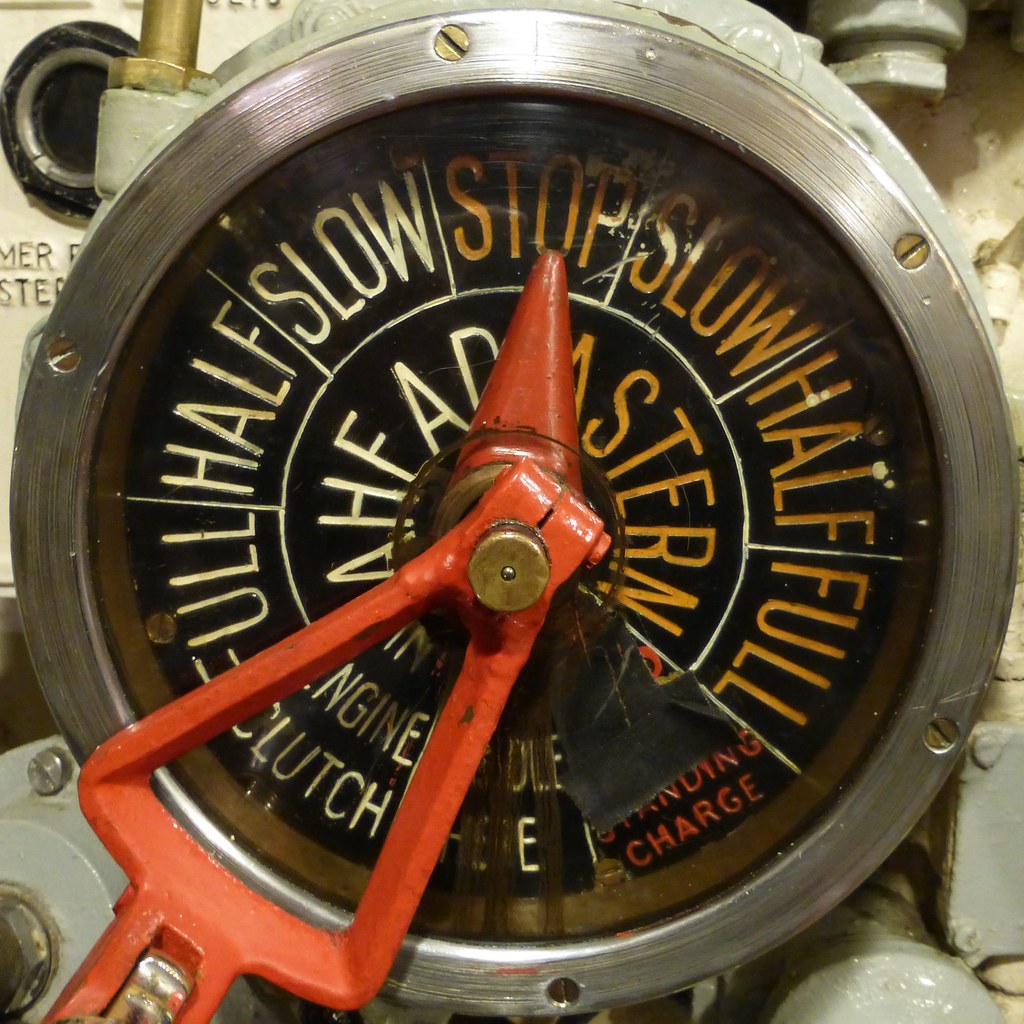The image depicts a detailed control gauge likely located on a large ship, set in an industrial indoor environment. At the center of the circular gauge is a prominent red lever designed to adjust various settings inscribed on the face of the gauge. The gauge itself is metallic silver with gold screws, and features a clear glass area displaying several labels in a clockwise sequence: "Stop" (highlighted in yellow), "Slow", "Half", "Full", "Charge", and "Engine Clutch." The lever is currently positioned at "Stop." Surrounding the gauge, multiple connected pipes appear to be secured with brass fittings and thickly painted, indicating their integration into the ship's broader system. The background includes additional piping and machinery components, adding to the industrial aesthetic. The use of colors in the image includes white, black, gold, silver, gray, red, and orange, enhancing the richness of this intricate maritime control setup.